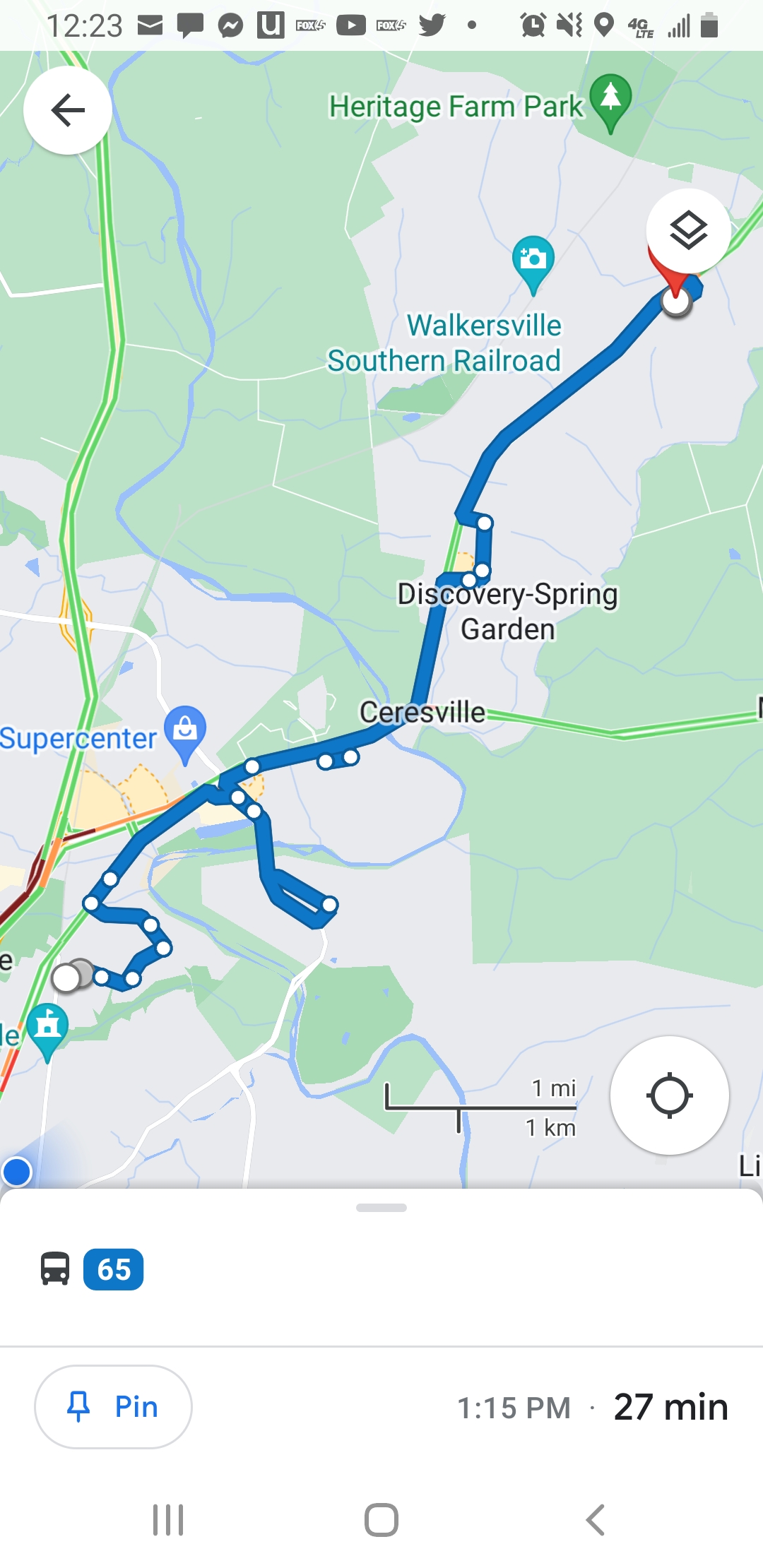Detailed Caption: 

A screenshot from Google Maps navigation on a smartphone shows a bus route from an unspecified starting point, located in the bottom left corner of the map, to the Walkersville Southern Railroad. Key landmarks are labeled on the map: Heritage Farm Park at the top, Walkersville Southern Railroad beneath it, and Discovery Spring Garden further down. Sayresville is marked towards the center of the map. To the left, a Supercenter is visible. The navigation icon below the map indicates that the journey will be made by bus, and the route is projected to take 27 minutes.